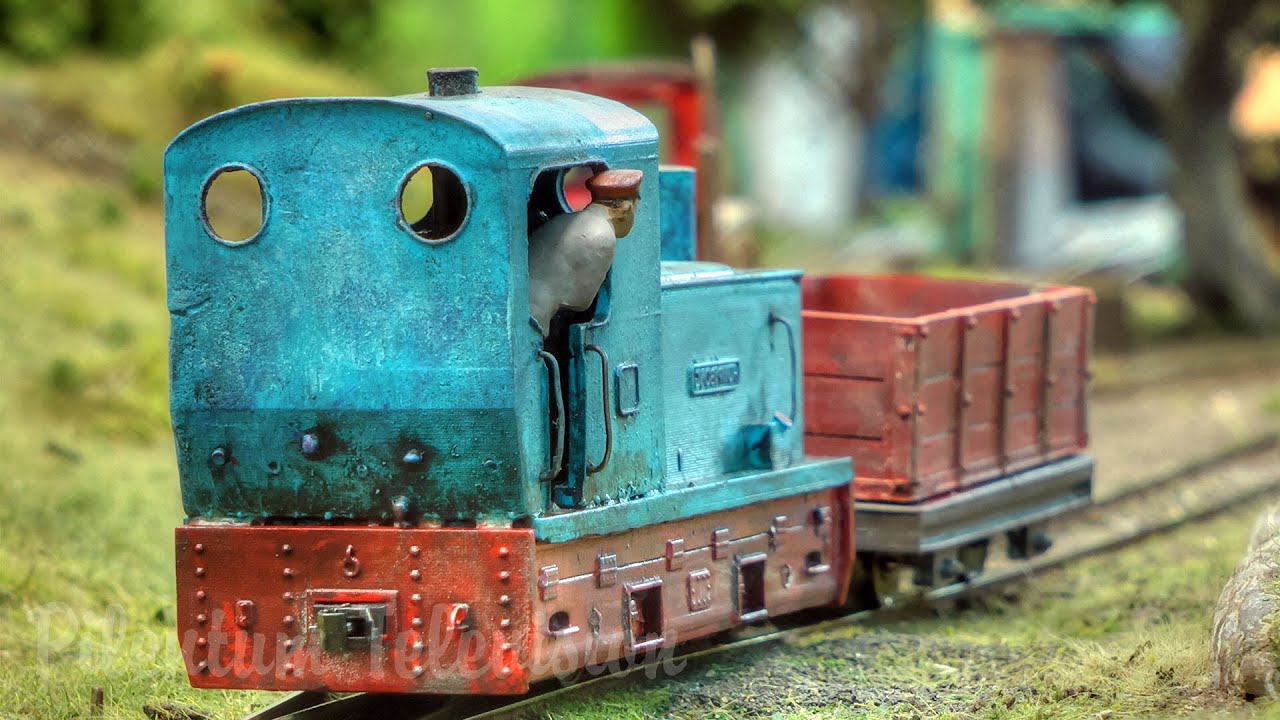This close-up photograph showcases an old, weathered toy train set placed outdoors on a miniature railway track. The toy train, reminiscent of vintage tin toys, features a red base and a cabin painted in a worn, metallic aqua blue with hints of rust. Rivets mark the rear, and hinges can be seen along the sides. The cabin, complete with a curved roof and two circular windows at the back, houses a figure of a conductor leaning out of the doorway. This conductor is detailed with a gray shirt and a flat red cap, peering across the train's length. Attached behind the engine, there is a single additional car with a black base and red paneled walls that are designed to resemble a container for cargo, though it stands empty.

The train tracks run from the bottom left to the right center of the frame, progressively blurring into the distance, creating a sense of depth. The background is out of focus, but it reveals a mounded grassy area, hinting that the train is set within a miniature village or playground. The entire scene evokes a nostalgic charm, emphasizing the train’s intricate details and the rustic outdoor setting. The blurred ambiance reinforces the spotlight on the toy train and its conductor, inviting viewers to step back into a simpler era of play.